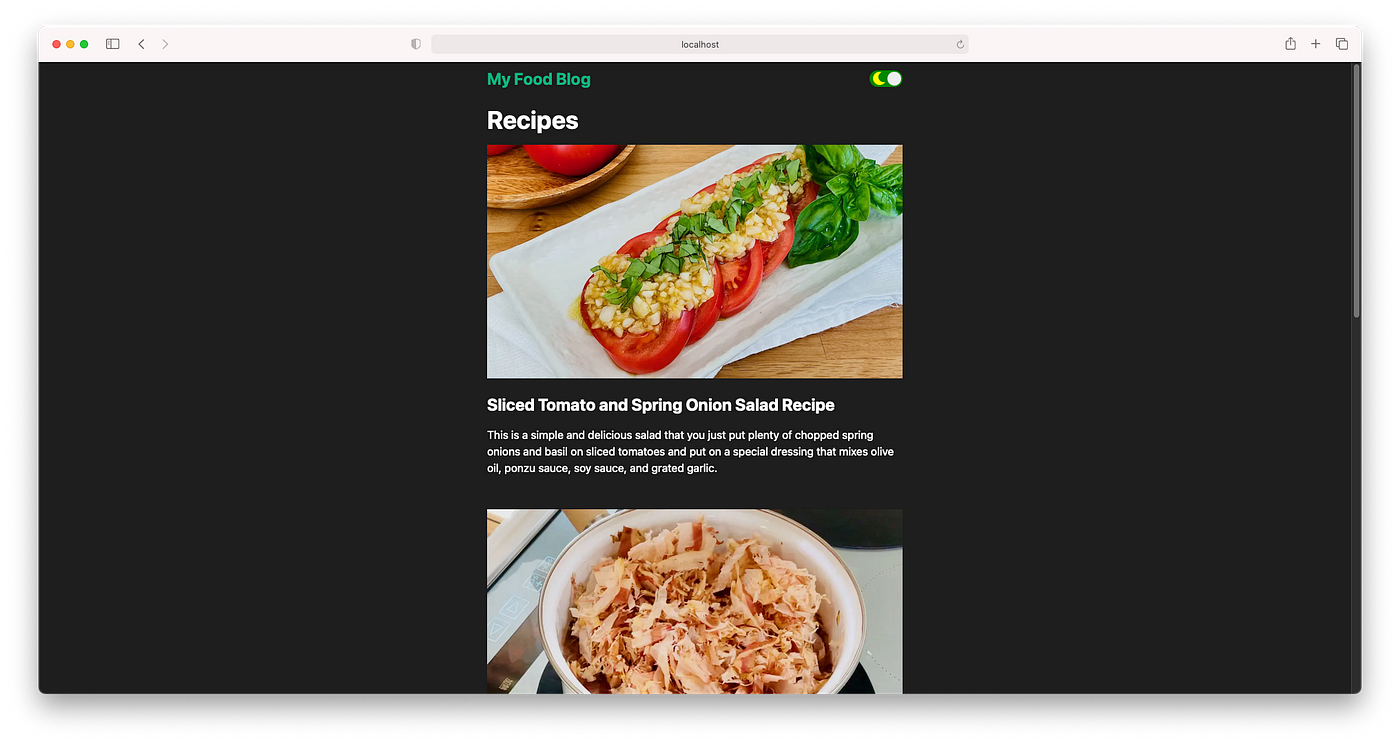The image depicts a blog-style website design. At the top, a white toolbar section is prominently featured, bordered at the top and housing several elements: three colored dots (red, yellow, green) in the upper left corner symbolize window control buttons. To their right are back and forward arrows, followed by a small shield icon and an address bar displaying "localhost." Adjacent to the address bar is a refresh icon, and further to the right are a plus sign for adding new tabs and a multi-window icon.

Beneath the toolbar, the page transitions into a black background, indicating dark mode, which corresponds with a toggle button displaying a yellow moon on a green background. The website title "My Food Blog" is prominently displayed in green text.

Below the title, an appealing image of tomatoes mixed with greens, possibly chopped spring onions and basil, is showcased alongside the text, "Slice Tomato and Spring Onion Salad Recipe." The accompanying description details a simple yet delicious salad recipe, emphasizing the use of chopped spring onions and basil on sliced tomatoes, dressed in a blend of olive oil, ponzu sauce, soy sauce, and grated garlic for a unique flavor profile.

Another image, likely of shredded chicken in a bowl, appears near the recipe content, adding visual appeal and context to the culinary theme of the blog.